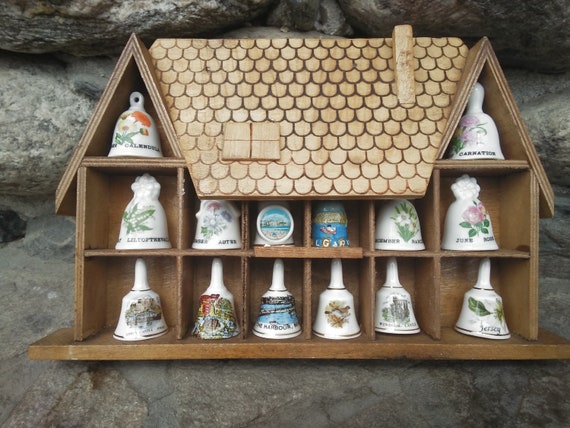The image depicts a miniature wooden house designed as a shelf, resembling a dollhouse but sized like a spice rack. This intricately crafted shelf, made of brown wood, includes a thatched roof with semi-circular tiles, a small wooden window, and a chimney. The interior features three rows of shelves separated into small compartments. Each compartment houses a white porcelain bell, each adorned with unique decorations ranging from flowers and plants to scenic paintings. Notable bells include one with red, yellow, and green leaves, another with purple flowers, and a central blue bell. Behind this charming knick-knack, a rocky gray background emphasizes the detailed artistry and colorful array of bells, creating a visually striking contrast. Some of the bells display names, possibly of plants, such as Jersey, Carnation, and Calanula, adding to the whimsical and personalized nature of the collection.